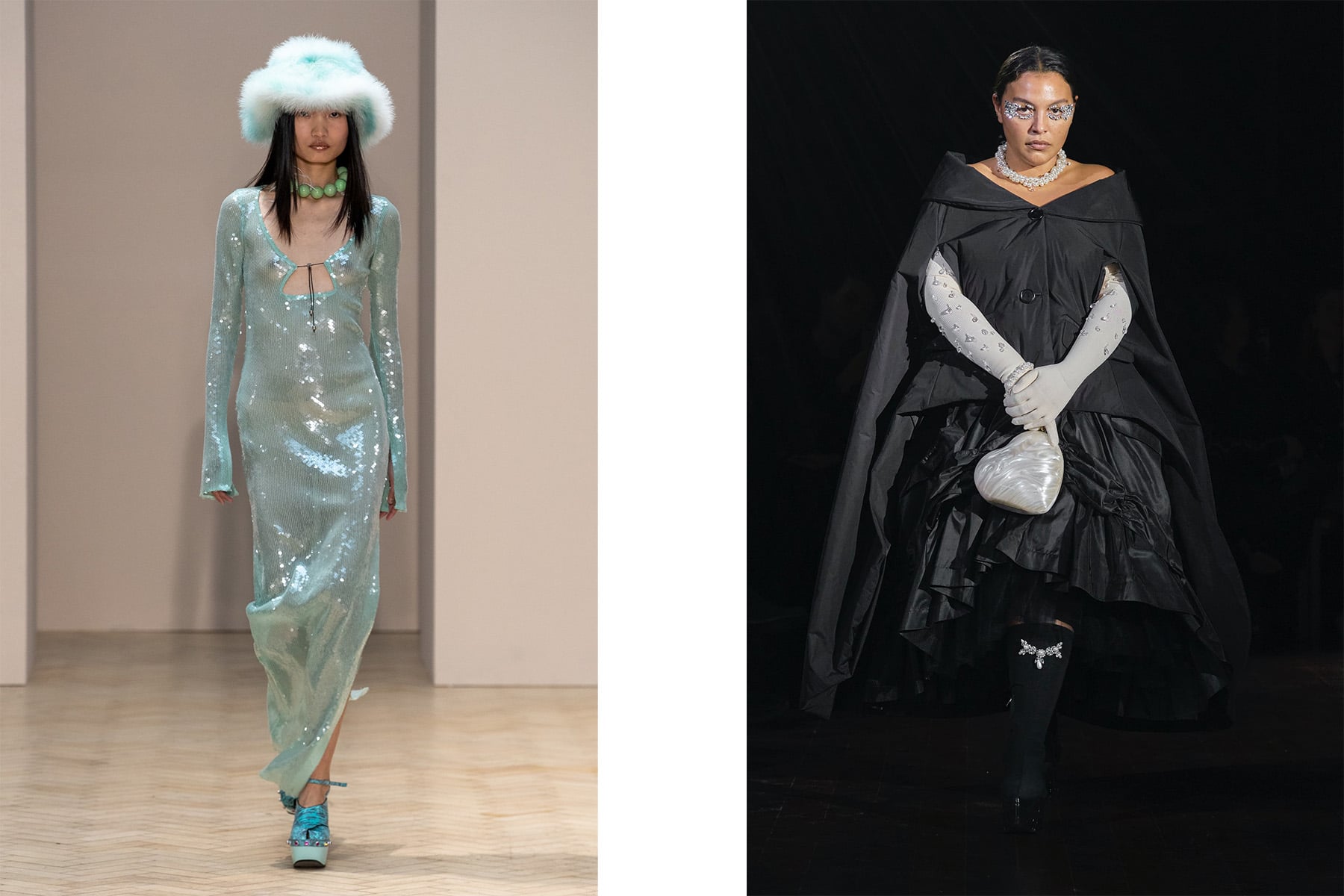The photograph is divided into two sections by a white vertical rectangle border. On the left side, there is an image of a runway model striding down what appears to be a fashion show runway. The background includes a tan or wooden texture, suggesting a hallway or backstage area. The model is a young, tall, and slender woman with long brown hair. She is wearing a transparent, glittery light blue or green dress that resembles a shower curtain and extends down to her bright blue neon shoes. She accessorizes the outfit with a fluffy light blue hat and a large green beaded necklace.

On the right side of the photograph, another woman, possibly the same model but older, is seen standing in front of a stark black background, enhancing the elegance of her attire. She is dressed in a very black, floor-length dress suitable for a serious occasion like a funeral. The dress appears to have a cape-like extension, but her long white-sleeved undergarment protrudes prominently, covering her hands. She carries a white heart-shaped purse or balloon on her lap and wears a striking silver or white circular necklace. Her eyes are adorned with intricate jewelry, and her hair is either short or pulled back. This composition emphasizes the contrast between the two different fashion looks and settings.